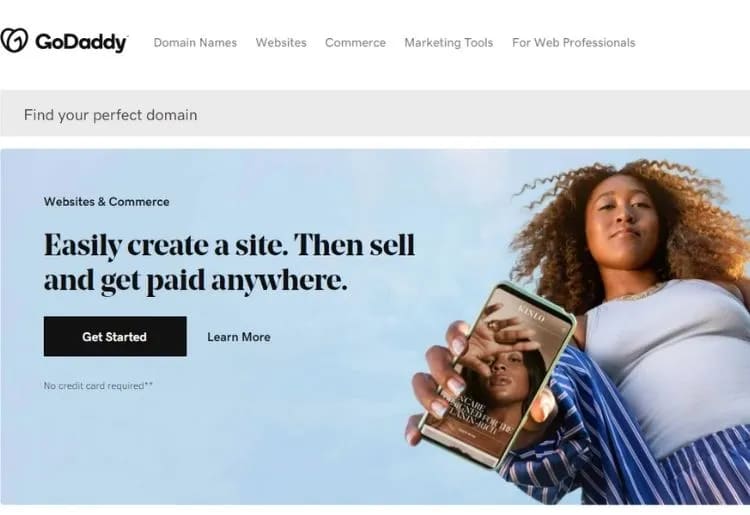The webpage displays the GoDaddy website, prominently featuring offerings for "Domain Names, Websites, Commerce, and Marketing Tools for Web Professionals" at the top. Below this, a search bar labeled "Find a Perfect Domain" in gray invites users to find their desired domain. A central banner emphasizes "Websites and Commerce" with a tagline that reads "Easily Create a Site, then Sell and Get Paid Anywhere." Below the banner, a black rectangular button with white text says "Get Started," alongside the note "Learn More, No Credit Card Required."

The background features a blue sky with scattered white spots, giving it an airy, sky-like appearance. Positioned prominently is a dark-skinned girl with brown curly hair, who is holding a smartphone. On the phone's screen, another girl is partially covering her face with her hand. The girl holding the phone is dressed in a blue and white outfit. The phrase "Learn More, No Credit Card Required" is repeated at the bottom of the page, highlighting the ease of starting with GoDaddy's services.